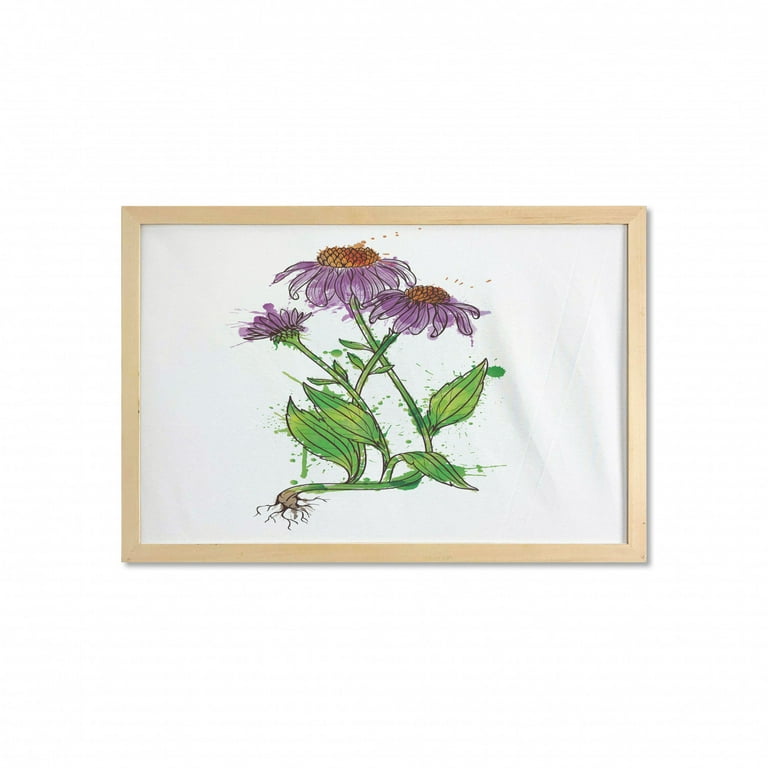The image showcases an artistic watercolor and ink composition, framed in a light wooden rectangular frame. The central subject of the artwork is an ink-drawn depiction of echinacea, commonly known as the purple coneflower. The watercolor painting appears on what looks like bunched up cloth, giving the surface a textured and crushed appearance. The flowers, with their purple petals and brownish-yellow cone-shaped centers, are accompanied by detailed green leaves and visible roots at the bottom left. The structure of the leaves features parallel venation typical of echinacea, with elliptical shapes that taper to a point. The composition is lively and slightly messy, with drips and dots of watercolor splattered outside the main outlines, enhancing its artistic charm. The piece is presented in a landscape orientation.